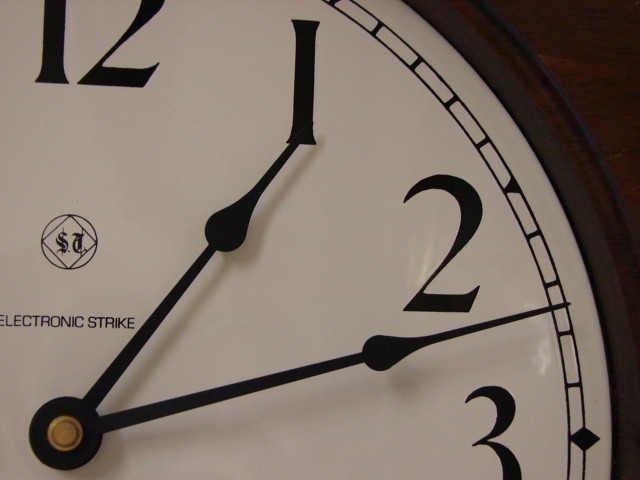A detailed segment of a traditional round clock is featured in this image, set against a muted brown backdrop. The visible section includes just over a quarter of the clock face, revealing numbers 12, 1, 2, and part of the 3, alongside sleek, black clock hands indicating the time as approximately 12 and a half minutes past one. The clock boasts a brown frame that complements the background, seamlessly blending into the setting. At the center of the clock face, the words "Electronic Strike" are clearly inscribed, nestled above a sophisticated emblem. This emblem comprises the initials "SJ" elegantly rendered in a flowing italic script, encapsulated within a combined circular and square logo.